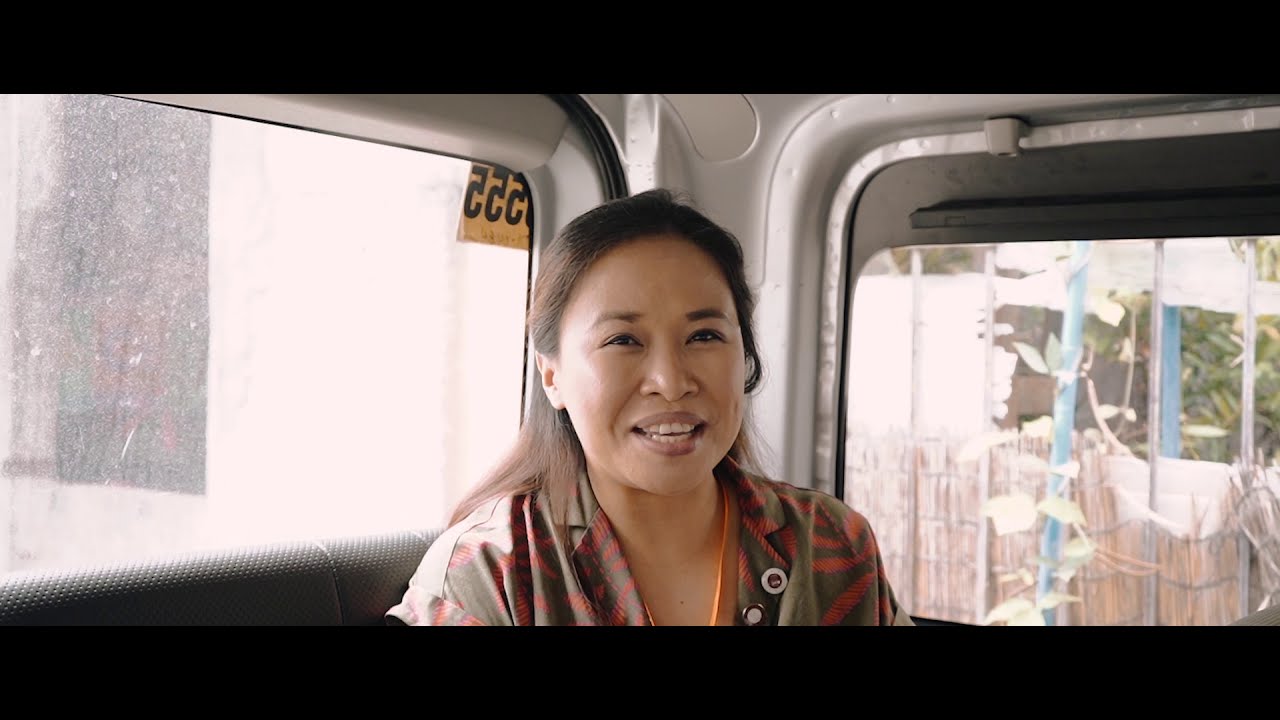This photograph captures a woman of apparent Asian descent, seated in the corner at the back of a vehicle, likely a bus, given the visible large windows to her left and right. Her dark hair is neatly pulled back from her face, accentuating her features, including dark eyes and a broad smile that reveals both her top and bottom rows of white teeth, complete with dimples. She exudes a sense of happiness and engagement, perhaps caught mid-conversation. 

She is dressed in a brown collared short-sleeve shirt decorated with red or orange leaf designs and some pins attached to her lapel. The vehicle's interior is predominantly white with gray seats, and a black strip runs across the top and bottom of the image. Notably, the window behind her bears a reversed "555" sticker with a yellow background. The exterior scenery seen through the right window includes a bamboo fence, greenery, and metal poles, whereas the view out the left window, though obscured by dirt, reveals a vague outline of a white building and a poster.